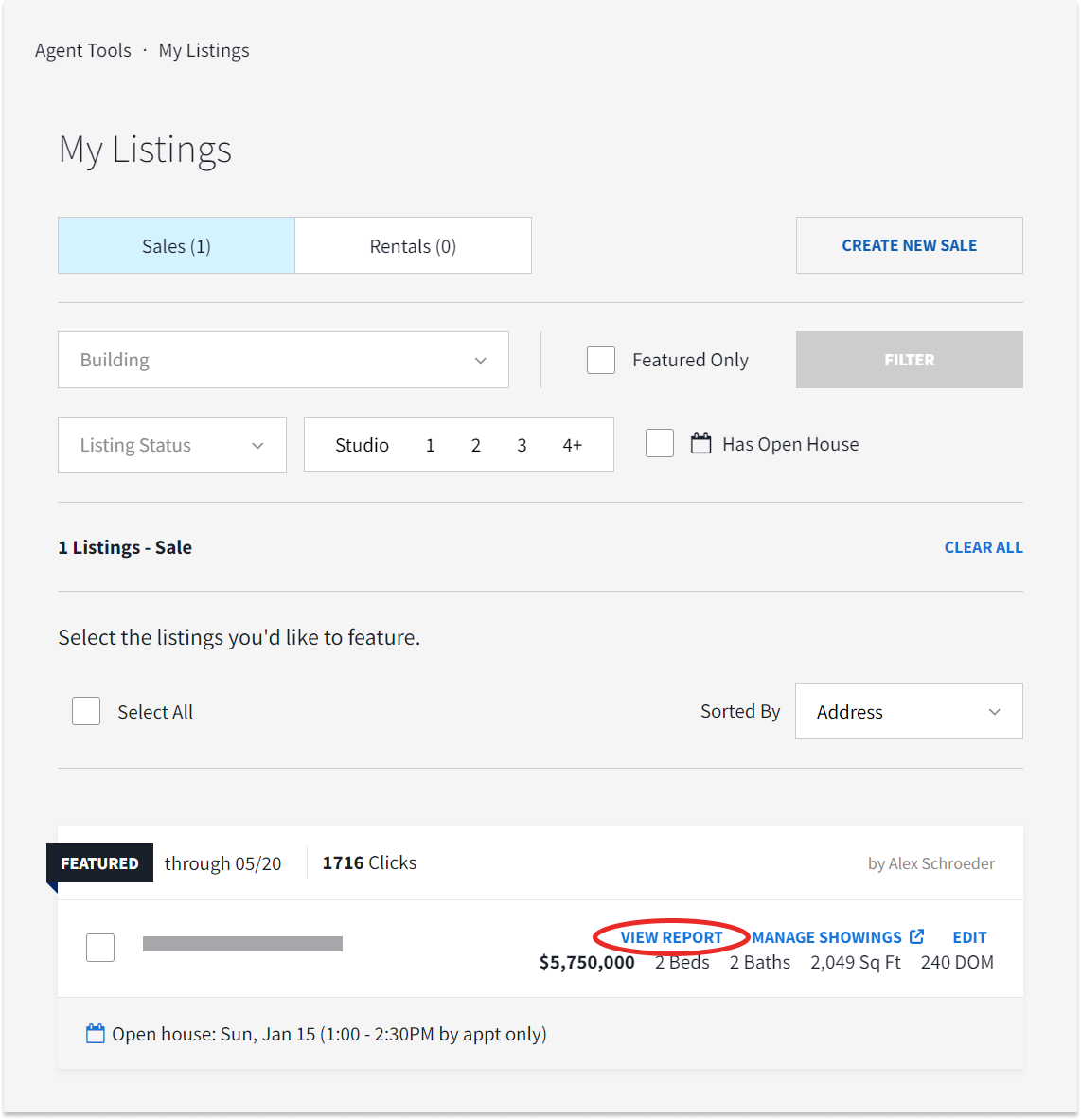The image features a light gray background with an interface showcasing agent tools and listing management. In the upper left corner, "Agent Tools" is displayed in black font, followed by "My Listings." Beneath that, the text "My Listings" appears in a larger font size. Two horizontal rectangular boxes are positioned side-by-side. The first box, in light blue, reads "Sales (1)" in black font, while the second box, in white, reads "Rentals (0)" in black font.

On the far right, a third horizontal box stands separate from the rest. This box is gray with blue uppercase text that reads "CREATE NEW SALE." A thin gray line divides the following section.

The subsequent section includes various horizontal rectangular fields with white backgrounds. The first field is labeled "Building" in gray font. Adjacent to this, a small checkbox is accompanied by the text "Featured Only." A gray button with the word "FILTER" in white all-caps text sits next to it. Below the "Building" field, another field is marked "Listing Status" in gray font with a dropdown menu option. Beside this, the term "Studio" is written in black, followed by options "1," "2," "3," and "4+" arranged horizontally. An empty checkbox is adjacent to the text "Has Opened House," which has an icon to its left. Another gray line separates this section from the next.

The next section begins with bold black text stating "One Listings-Sale," and to the right, in blue uppercase letters, "CLEAR ALL." A horizontal line follows. Then, black text reads, "Select the listings you'd like to feature." Below this, an unchecked box is labeled "Select All." Next to this, there's a dropdown menu in a white horizontal box labeled "Sorted By," displaying "Address." 

At the bottom, another white horizontal box contains a black horizontal rectangle on the upper left corner with "FEATURED" written in bold white font. Beside this, it states "Through 05/20," followed by "1716 Clicks." Farther to the right, it reads "By Alex Schroeder." On the left, an empty checkbox is present, followed by a thick gray horizontal line. 

To the right, categories in turquoise all-caps letters are visible: "VIEW REPORT" (circled in red), "MANAGE SHOWINGS," and "EDIT." Underneath, the details "$5,750,000," "2 beds," "2 baths," "2,049 sq ft," and "240 DOM" are listed. In the off-white/light gray area to the right, there is an icon of an open house and text that reads "Open House: Sunday, January 15th (1:00 to 2:30 p.m.) by appointment only."